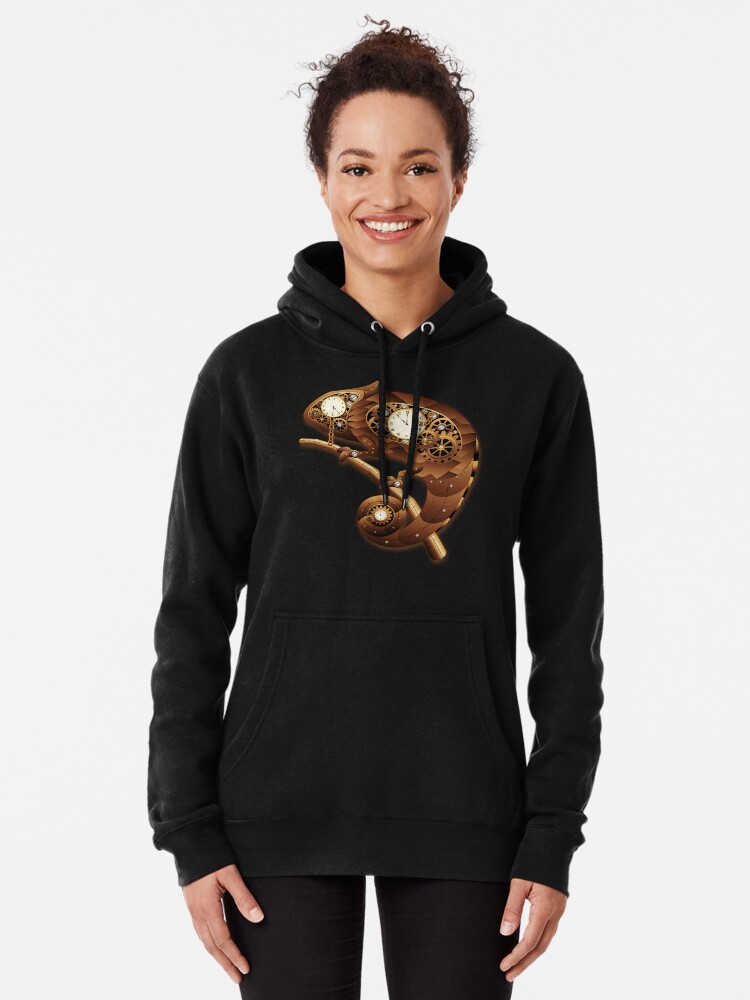This is a professionally posed, full-color, vertically rectangular photograph taken indoors using artificial light. The image features a light-skinned black woman with brown eyes and brown, frizzy hair, tied back with strands sticking up wildly. She is smiling warmly, showing her teeth, and looking straight at the camera. Her hands are relaxed at her sides. She is dressed in a dark blue or black long-sleeve hoodie sweatshirt with the hood down and matching black pants or leggings.

The central focus of the hoodie is a detailed, steampunk-style design of a chameleon or gecko. The animal, positioned centrally on the hoodie, is rendered in brown and bronze tones. It features intricate elements such as white clock faces on its head, body, and tail, and is adorned with various gears and mechanical components. The chameleon is depicted clutching a thin brown stick within the design. This detailed portrayal emphasizes the artistic and mechanical aesthetic of the steampunk genre. The background of the image is a very light or off-white color, with no additional text or borders, ensuring the focus remains entirely on the model and the intricately designed hoodie.